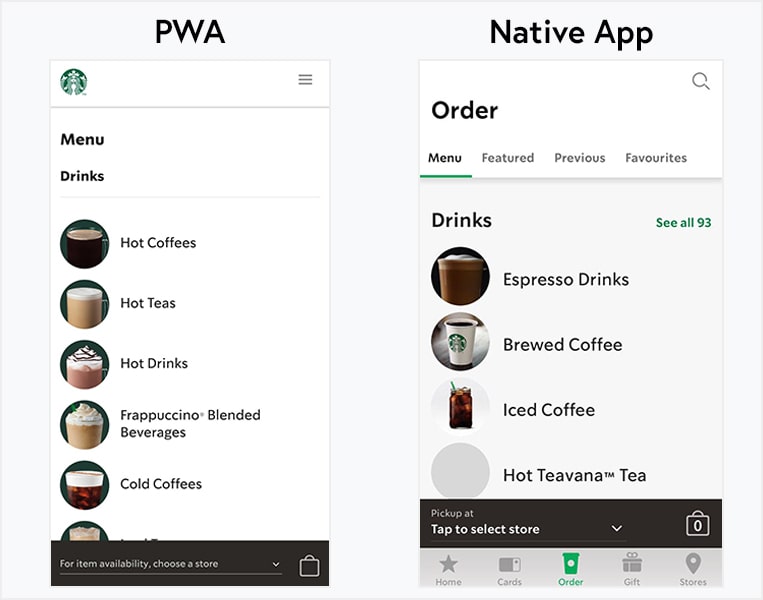Detailed Caption:

A detailed screenshot of a Starbucks menu displayed on a mobile app shows a wide variety of beverage categories including PWA menu drinks, hot coffees, hot teas, and hot drinks, each accompanied by corresponding images. The categories also feature Frappuccino blended beverages and cold coffees. Although the top portion of the image is visible, the text is obscured. Evident in this section is what appears to be either iced coffee or a frappuccino, identifiable by visible ice. The interface indicates that item availability depends on the selected store, and there is an option beside this for selecting the number of items, represented by a shopping bag icon. 

In another screenshot, the native app's order menu highlights various options such as featured items, previous favorites, and a menu underlined in green. The extensive menu offers drinks, espresso drinks, brewed coffee, iced coffee, and hot Teavana tea. Notably, the Hot Teavana tea category lacks an image. A prompt at the top right corner instructs users to "see all 93" items, displayed in green, contrasting with the black text elsewhere. Options at the top include "pickup at" with a prompt to tap to select a store, and a shopping bag icon showing zero items. At the bottom of the screen, navigation options are available in a horizontal menu, including "home," "cards," "order" (highlighted in green), "gift," and "stores," with the remaining options in gray.